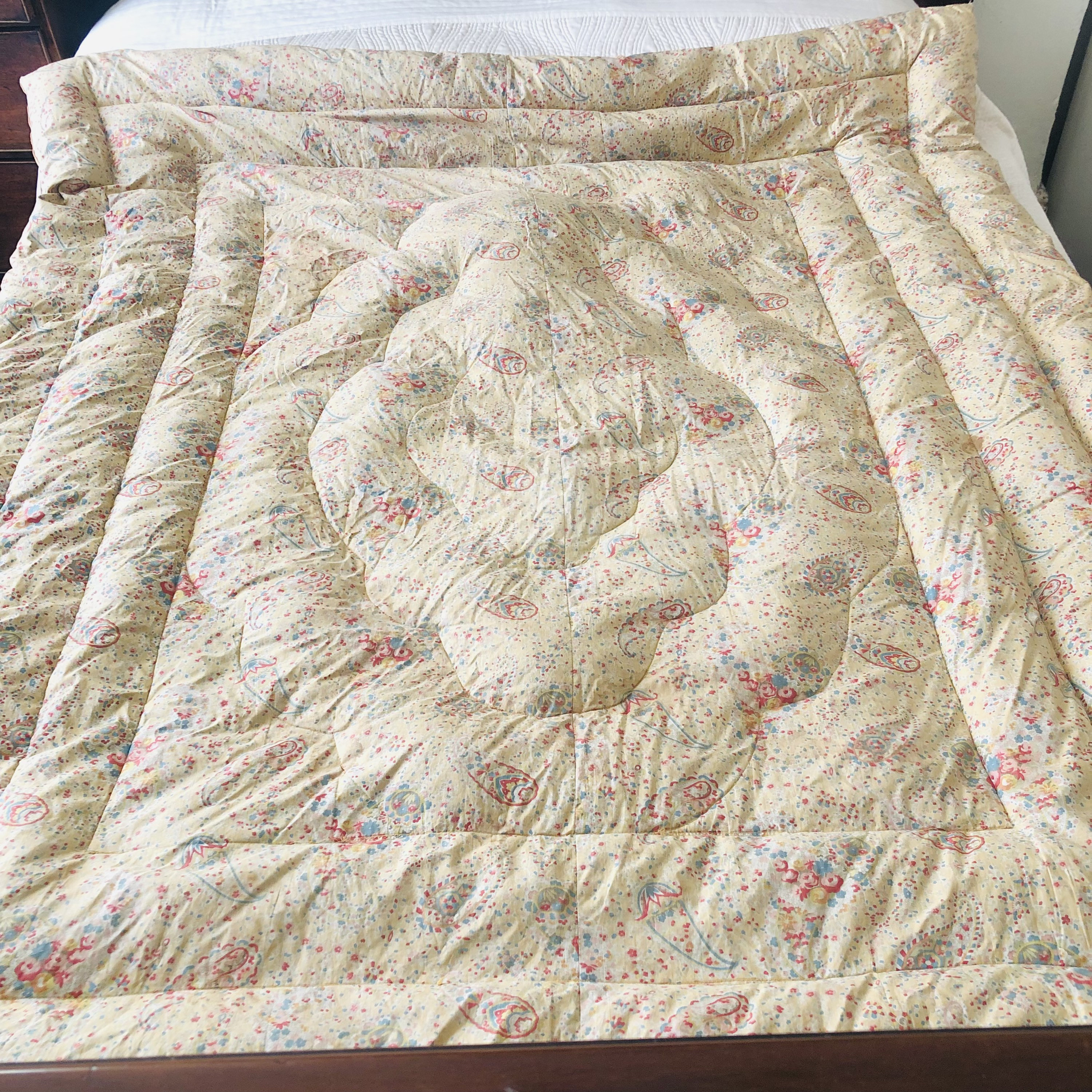The square-shaped photograph, taken indoors in a bedroom, focuses on a luxurious, eiderdown quilt that dominates the scene. The quilt, suitable for a double bed, is spread out and central to the image. It features a light, almost cream-yellow background adorned with delicate, dainty floral prints in shades of blue, pink, and a hint of green. The intricate floral pattern covers the entire surface of the quilt, adding a touch of elegance to the room. The stitching on the quilt is detailed, starting with a box stitch that creates rectangles of progressively smaller sizes toward the center, culminating in a central stitch that resembles a rose. This combination of layers and patterns adds depth and texture to the quilt. The backdrop includes a white mattress partially visible, along with wooden furniture that suggests drawers or a dresser on the left side of the image, enhancing the cozy bedroom ambiance.